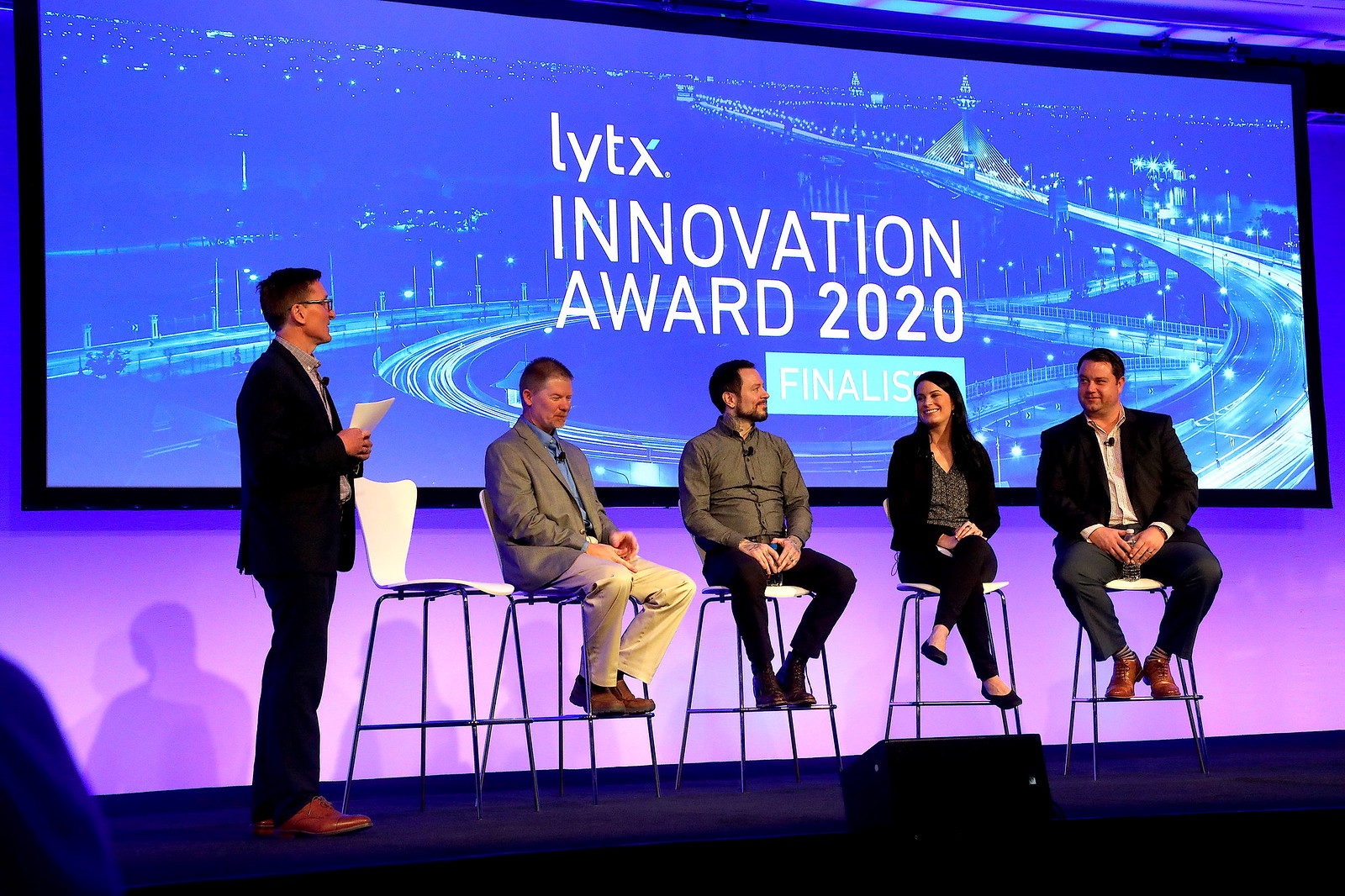On stage at what appears to be the LYTX Innovation Award 2020 event, a group of five individuals engaged in what looks like a keynote presentation or panel discussion. The backdrop, a large, illuminated screen, showcases a nighttime highway scene with sparkling lights, reinforcing the theme of innovation. The words "LYTX Innovation Award 2020" are prominently displayed above the imagery, with a faint purple hue casting shadows on the wall beneath.

Seated on sleek white chairs with silver legs, four of the five participants are arranged from left to right. The scene begins with a standing man on the far left, dressed in a black suit with short black hair, glasses, and a piece of paper in hand—possibly the emcee. His polished appearance is complemented by leather shoes. Next to him is an empty chair, followed by a gentleman in business attire featuring a gray suit, blue shirt, khaki pants, and orange and leather shoes, who faces downward thoughtfully.

Continuing right, the next seated man sports a gray shirt, black pants, and a full beard, his hands positioned openly near his lap while he looks to his right. Adjacent to him sits a smiling woman with long black hair cascading past her shoulders. She wears a black jacket, black pants, and V-neck shirt, crossing her legs to display black shoes. Finally, the last chair houses another man in black attire—jacket and pants—with a light-colored shirt and leather shoes. A notable detail is the black box positioned directly in front of the seated individuals on the stage floor, adding to the organized yet dynamic setup of this professional gathering.